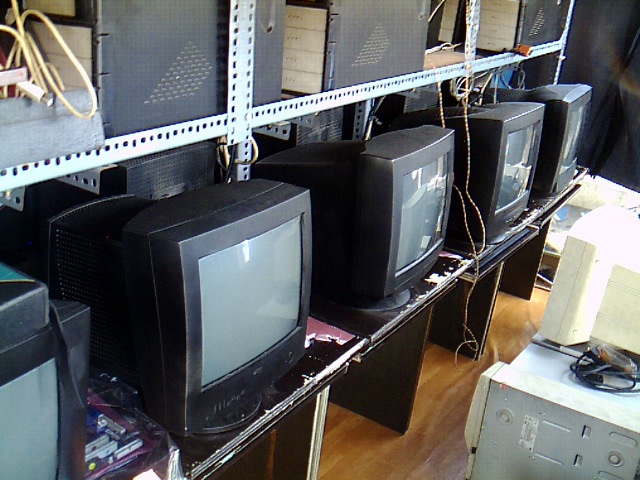The image depicts a room resembling a storage area or a makeshift display setup, showcasing a collection of old technology. Central to the scene, a sturdy steel shelf with a wooden surface holds five identical vintage CRT computer monitors, each encased in black plastic with light gray convex screens. Above these monitors, three black, boxy devices rest, possibly old modems or external hard drives, featuring wooden sides and trapezoidal fronts, slightly obscured by hanging wires. The shelf stands on a light wooden floor, which has subtle darker lines running through it. To the right of the black monitors, there is an additional setup: a white CRT monitor facing away, perched on a gray steel cabinet, further accentuating the technological relics on display. The overall color scheme is predominantly monochromatic, with the black and gray monitors contrasting against the light floor and steel shelving, unified by the backdrop, which appears dark and minimalistic.